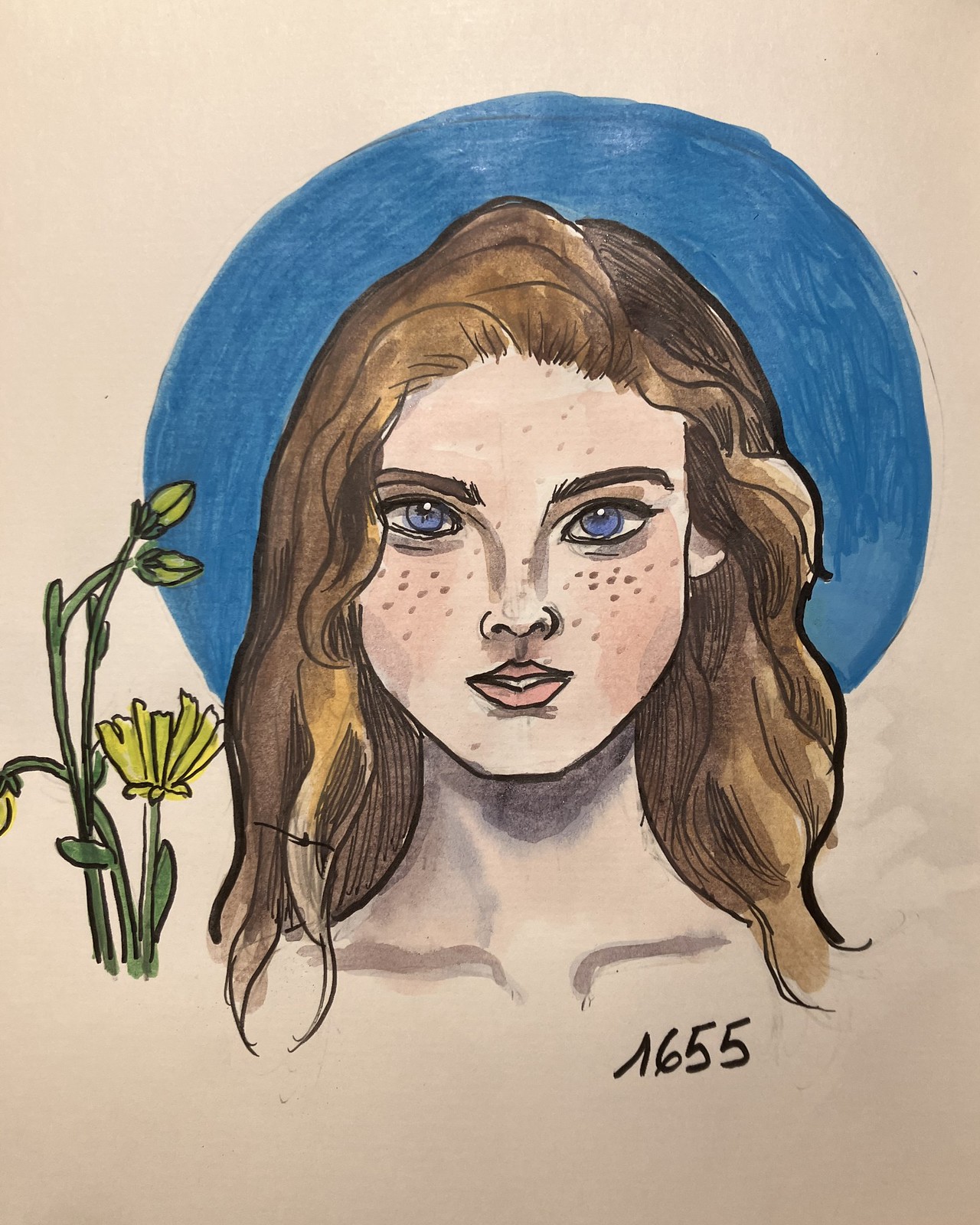This detailed watercolor painting, executed on an off-white piece of paper, portrays a young girl facing forward. She wears a distinct blue sun hat with a large brim that sits on the back of her head. Her shoulder-length, slightly wavy hair is a mix of light brown and reddish tones. She has expressive blue eyes, dark eyebrows, and a sprinkling of freckles across her cheeks and nose. Her lips are a soft pink, and her mouth is slightly open, revealing a hint of an expression. The painting captures her neck and collarbones, with the remaining details fading away below that.

To the left of the girl, a small cluster of flowers is depicted with delicate attention to detail: a yellow flower in full bloom accompanied by two taller stems housing yellow buds. In the lower right corner of the artwork, the artist has signed it with the characters "A655" in black marker. The entire background of the painting maintains a flesh-toned hue, completing the harmonious composition.